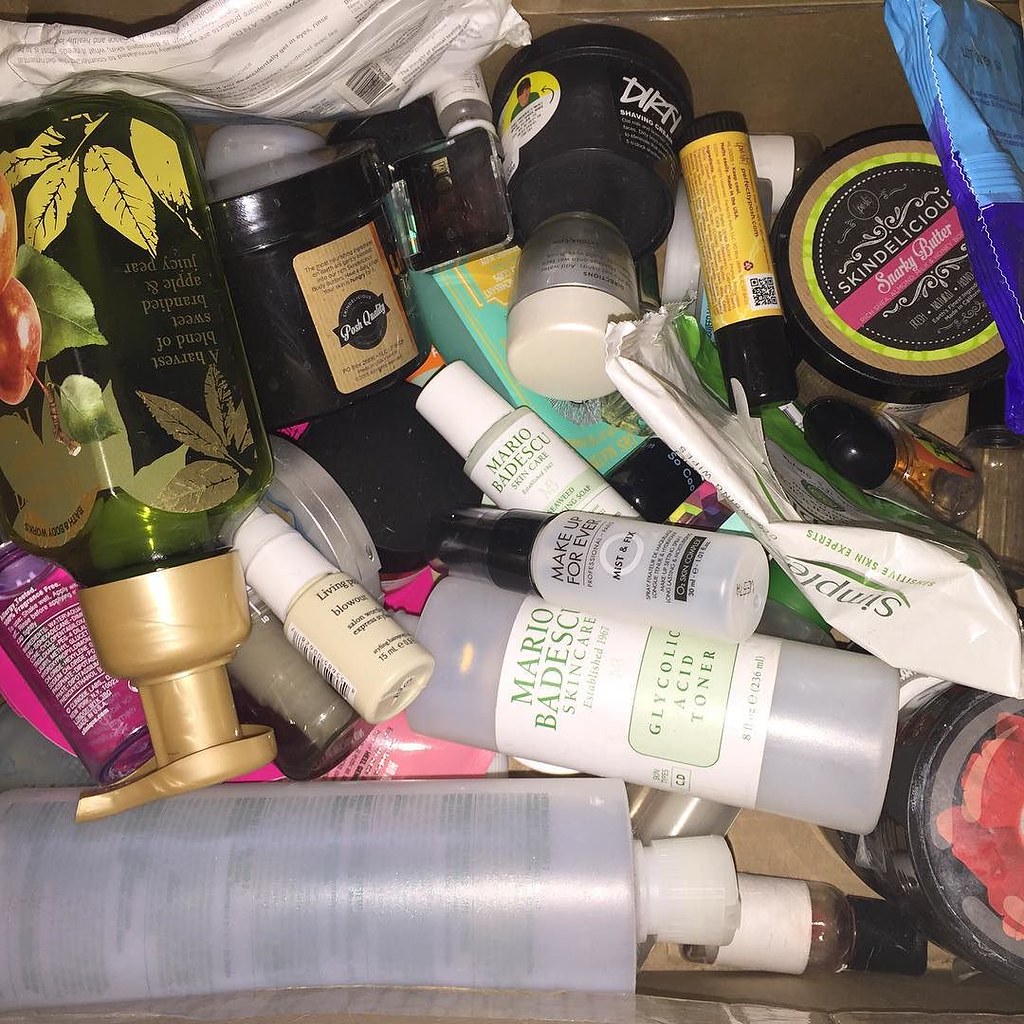A top-down photograph captures a somewhat shallow drawer filled with an eclectic assortment of skincare and beauty products. The drawer is a chaotic, yet intriguing, display of various bottles and containers, ranging from small sample sizes to larger jars. Among the collection, one can identify a glycolic acid toner, several makeup items, and a variety of skincare products. Some bottles feature pump dispensers for easy application, and one bottle is noticeably upside down. A prominently labeled "Harvest Blend of Sweet Branded Apples" and a large container of "Skin Delicious Snarky Butter" stand out amidst the diversity. The drawer showcases a mix of professional-grade skincare and health products in an array of colors, shapes, and materials, including plastic and glass packaging, making it a treasure trove of beauty essentials and treatments.